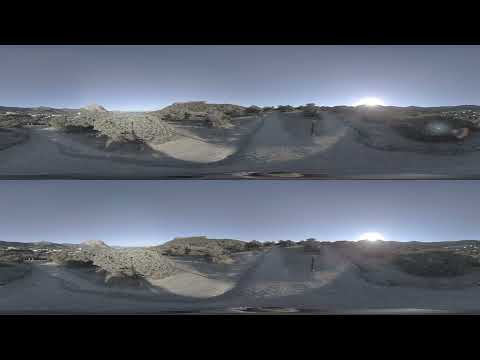The image is a landscape-oriented color photograph featuring a sandy dune landscape split into two identical horizontal sections, one above the other, separated by solid black lines at the top and bottom. The scene is captured in a panoramic style with photographic representationalism and special filters applied. The image depicts a wide sandy hill, appearing tan with shadowed areas, set against the backdrop of a setting or rising sun, creating a bright yet dusk-like sky with shades of light blue, gray, and white. Along the horizon, a few overgrown bushes and trees display a whitish-green hue. The terrain includes two parallel dirt roads running through the center, hinting at a possible park or walking area. The overall visual composition emphasizes the serene, natural beauty of the sandy dunes with sporadic greenery, adding a touch of lifelike vibrancy to the landscape. The absence of text in the image ensures that the focus remains on this tranquil outdoor scene.